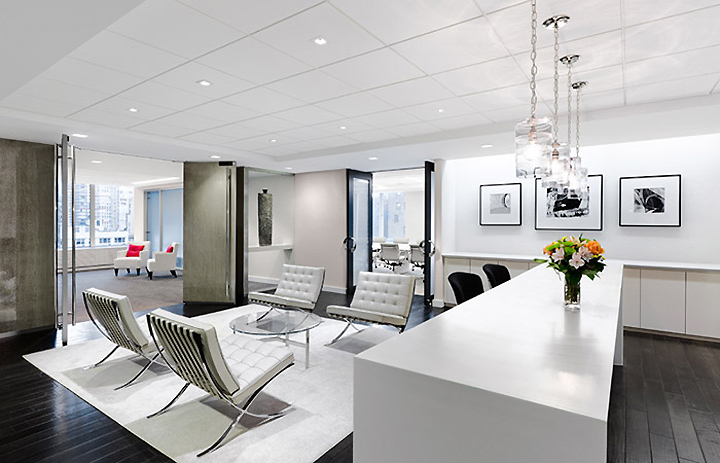The image captures a modern indoor office space or stylish apartment with a predominately white and sleek design. The room boasts white walls and a white square-paneled ceiling, illuminated by a combination of recessed lighting on the left and multiple glass globe ceiling lights on the right. Below the globe lights is an exceptionally long white table, adorned in its center with a vibrant bouquet of white and orange flowers, flanked by ergonomically designed black chairs. To the right of this setup, three square picture frames with black borders adorn the wall, while below them, a counter space with numerous cupboards adds functionality to the aesthetic.

The centerpiece of the room is a round glass coffee table placed on a large white rectangular rug. Around the coffee table are four white chairs with silver backs and feet, appearing both modern and slightly resembling lawn chairs due to their design. The flooring transitions from wooden panels on the right, with gray tones blending into darker hues toward the left side of the image.

On the left side, we observe an entrance leading into another room furnished with white chairs featuring red throw pillows and gray carpet flooring, illuminated by natural light streaming through a large open window, indicating daytime. The back-center of the image reveals a pair of black-framed doors with frosted panes, opening into another room that seems to serve as a meeting space, fitted with a table and multiple chairs. This caption amalgamates the repeated and distinct elements described while emphasizing the room’s modern, clean, and airy atmosphere.